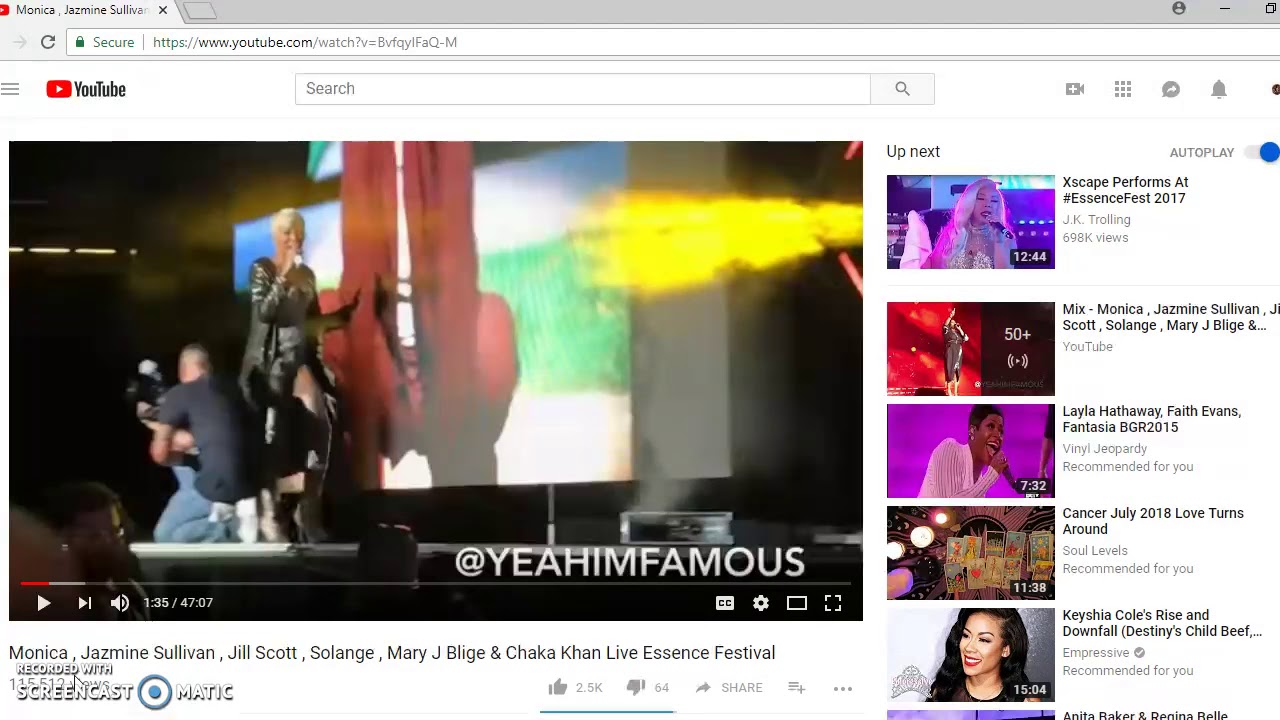The image is a screenshot of an old YouTube interface, showcasing various video titles and elements. The highlighted video appears to be titled "Yeah I'm Famous," possibly produced by the referenced tag. The video description lists a star-studded lineup including Monica Jasmine Sullivan, Jill Scott, Solange, Mary J. Blige, and Chaka Khan, performing live at the Essence Festival. Additionally, there is a visible watermark from "Screencast-O-Matic" on the screenshot. Various other video titles and events are also mentioned, such as "Xscape performs at Essence Festival 2017," and performances by "Layla Hathaway," "Faith Evans," and "Fantasia" from the 2015 Essence Festival. There is also a video from 2018, capturing a nostalgic look at YouTube’s previous layout.